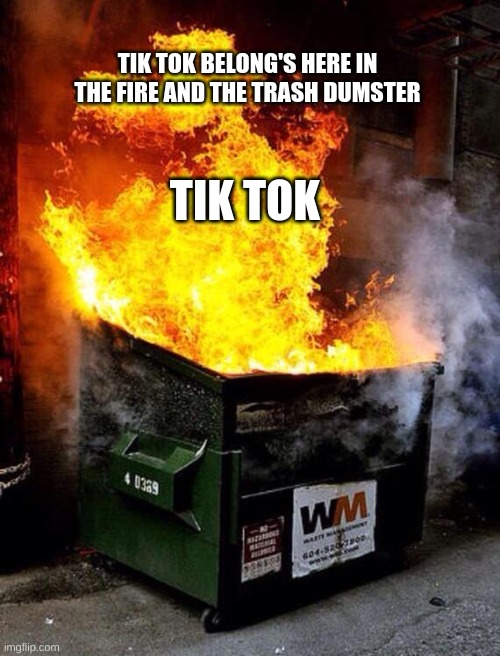The photograph depicts an outdoor scene featuring a prominent green dumpster positioned on a city street, likely behind a commercial building. The dumpster belongs to the Waste Management company, as indicated by a large white sticker with the letters "WM" and the company name, though the accompanying phone number is unreadable due to heavy wear. The dumpster is ablaze, with intense orange, red, yellow, and white flames and smoke pouring out, suggesting a fiery inferno. The dumpster is equipped with small black caster wheels and side brackets for truck pickup. Imposed over the image in bold white text are the words: "TikTok belongs here in the fire and the trash dumpster. TikTok," conveying a clear anti-TikTok sentiment. The varied colors and intense flames dominate the bottom half of the image, with additional details like pipes and potential building structures faintly visible in the background. The text and the dramatic blaze create a striking and vivid commentary.